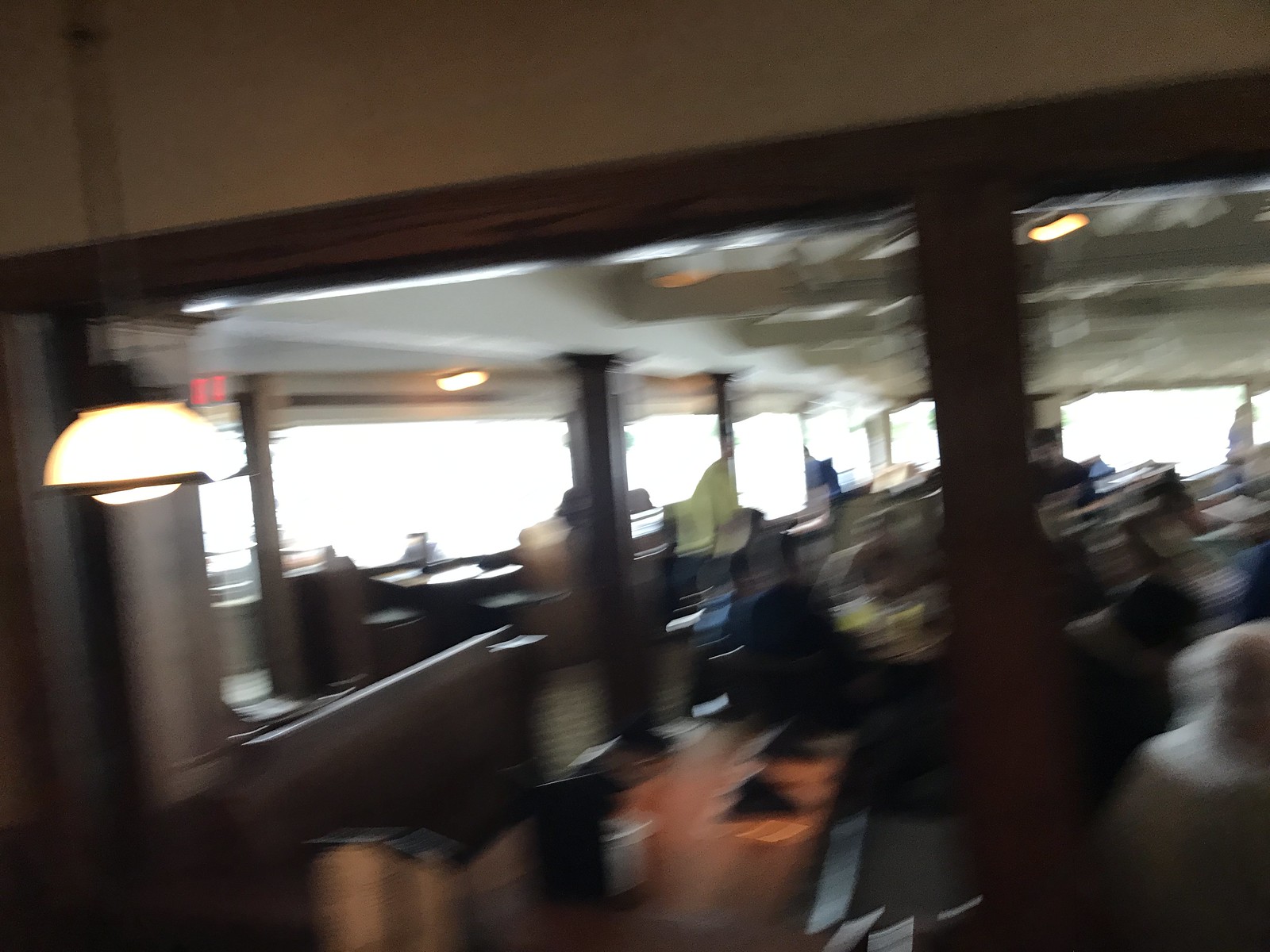The image depicts an out-of-focus interior that is likely a restaurant. The scene features several tables and wooden booths or seats, all adorned with various items such as napkins or dispensers. Overhead, there are multiple lamps hanging from the ceiling, including a white light fixture on the left-hand side suspended by a black cable or chains, trimmed in dark brown. The flooring appears to be brown hardwood, and the architectural detailing includes dark brown wooden trims and possibly columns or posts supporting different sections of the ceiling.

Towards the top of the image, a white wall with dark brown trim is visible, and there are indications of yellow and red lights in the ceiling, adding to the ambient glow. The background reveals several windows, with sunlight streaming in, creating patches of light across the space. A possible archway framed in wood suggests an entrance to another room. The lower part of the image displays a potential figure in white in the right-hand corner and another in a black shirt more centrally. Despite the image's blurriness, the ambiance and structure of a bustling dining space are evident, complete with scattered details and a softly lit environment.